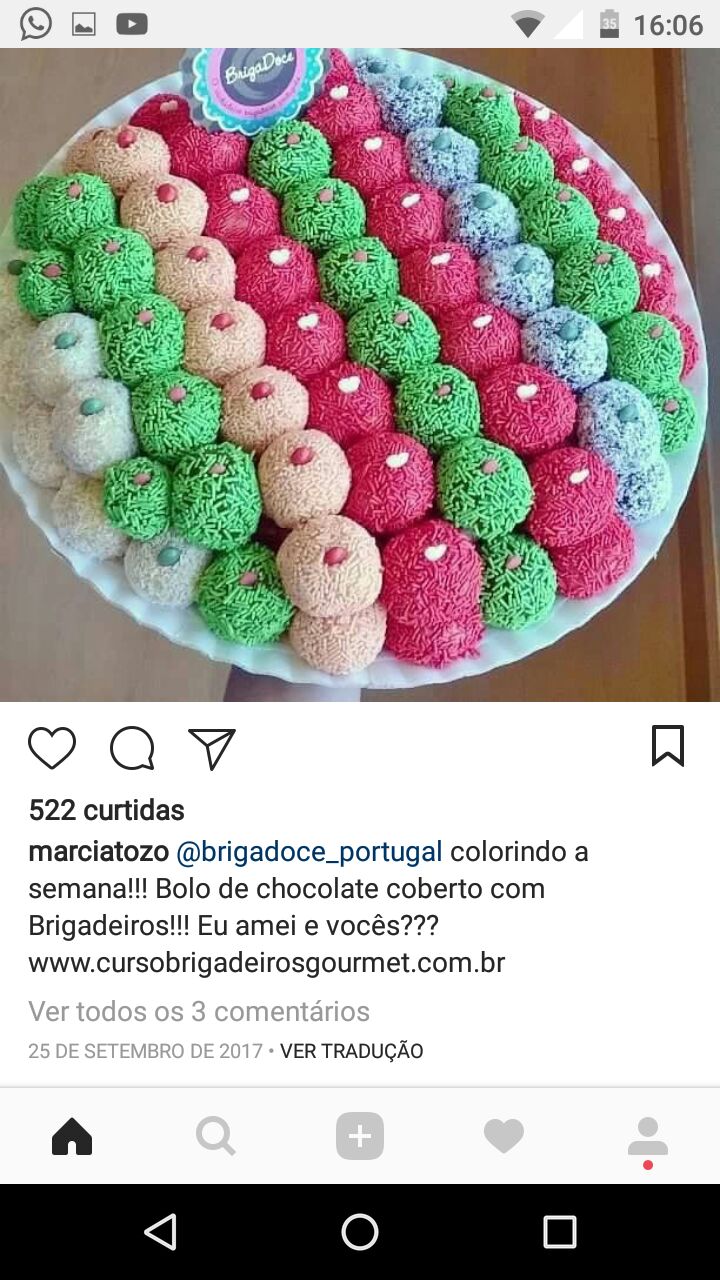This Instagram post, dated September 25th, 2017, features a detailed photograph of a beautifully arranged plate of colorful, sprinkle-covered sweets that resemble traditional Indian confections. The plate itself is white with a scalloped edge, adding an elegant touch to the presentation. The sweets are meticulously organized in two layers, each layer displaying stripes of vibrant colors. 

Starting from the left, the sequence begins with white, followed by pale blue with darker blue dots, then green with pink dots, light pink with darker pink, red with white, green with gray, another set of pink with white, blue with dark blue, green with brown, and finishing with pink with white. The careful arrangement of colors and layers creates a visually appealing and delicious-looking display. Below the image, the text is written in Spanish, adding an international flair to the post.